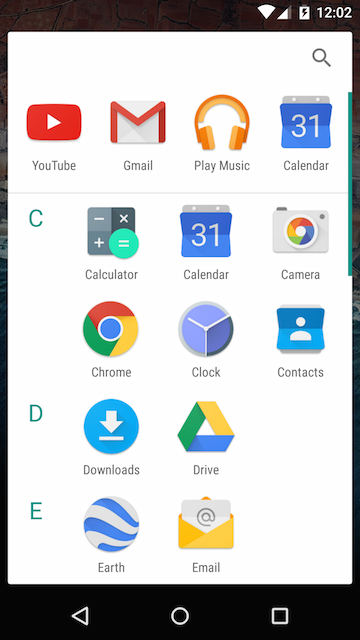The image depicts the home screen of an Android phone. Displayed prominently are various app icons organized in alphabetical order. At the top of the screen is the status bar, indicating a Wi-Fi connection, a charging battery with a percentage indicator, and the current time, which reads 12:02. 

The first row of icons features, from left to right, YouTube, Gmail, Play Music, and Calendar. Beneath this row is a label "C," followed by icons for Calculator, Calendar, and Camera. The subsequent row includes icons for Chrome, Clock, and Contacts. The fourth row, labeled "D," includes Downloads and Drive, identified by its cloud-like symbol. The final labeled row "E" contains the icons for Google Earth and an email application.

Positioned at the very bottom of the screen are the navigation controls: a circular Home button in the center, a triangular Back button to the left, and a square representing the Recent Apps function to the right.